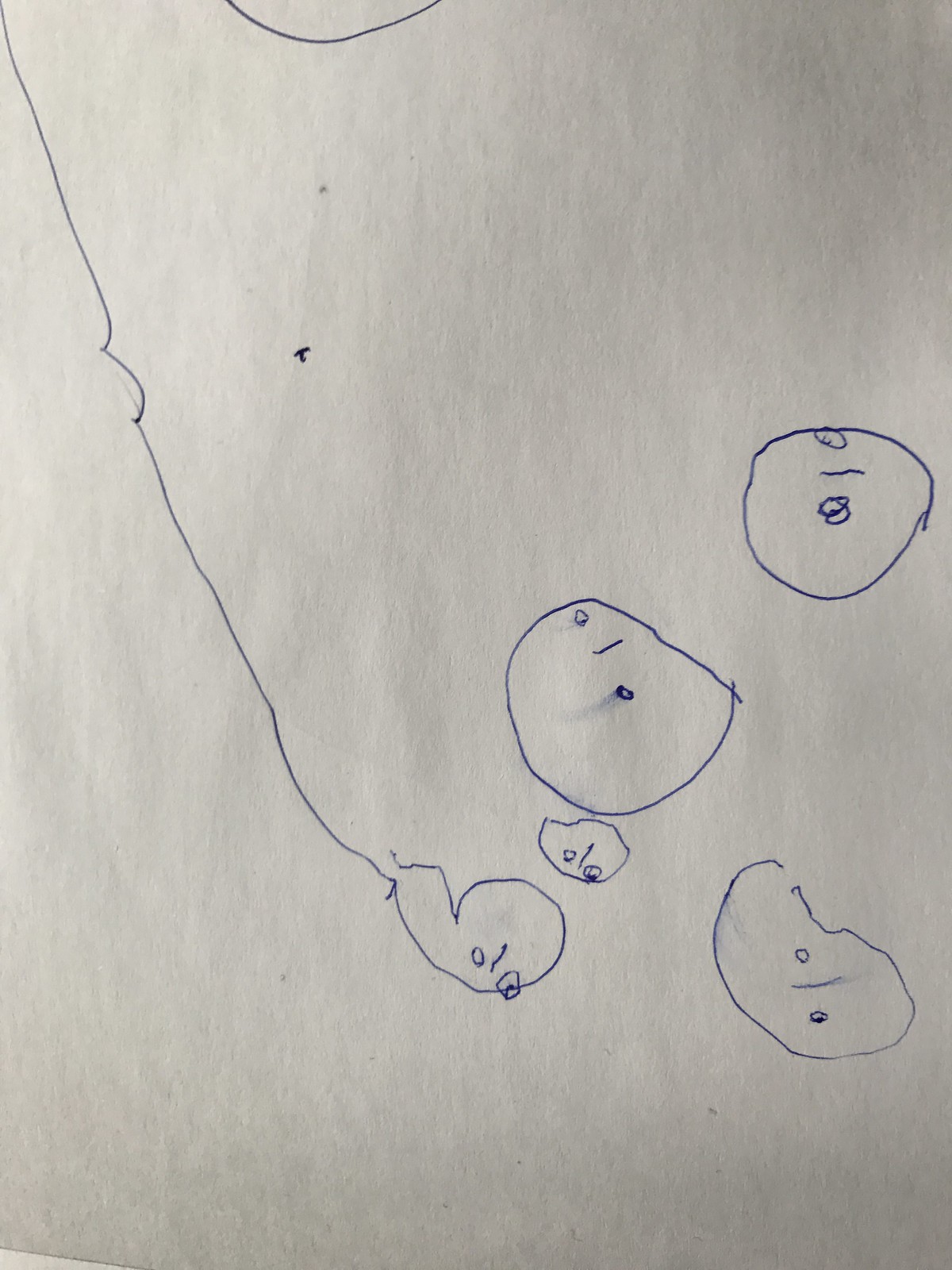The image features a white piece of printer paper with a drawing made in blue pen. The drawing appears to be slightly cut off but shows the lower half of a circle at the bottom. To the left, there's a line resembling a fishing pole with a fish hooked at the end. The hooked fish is detailed with two eyes and a nose but lacks a mouth. In addition to this fish, there are four other similar figures scattered across the page, each displaying eyes and a nose but no mouth, creating a cohesive visual theme. A blue dot is located in the center of the paper, which might represent fish food or bait, or it could be a stray mark from the pen. The orientation of the fish suggests they are either upside down or turned sideways. A small corner of the paper is visible at the bottom left, and the entire setup appears to be placed on a white table or desk.